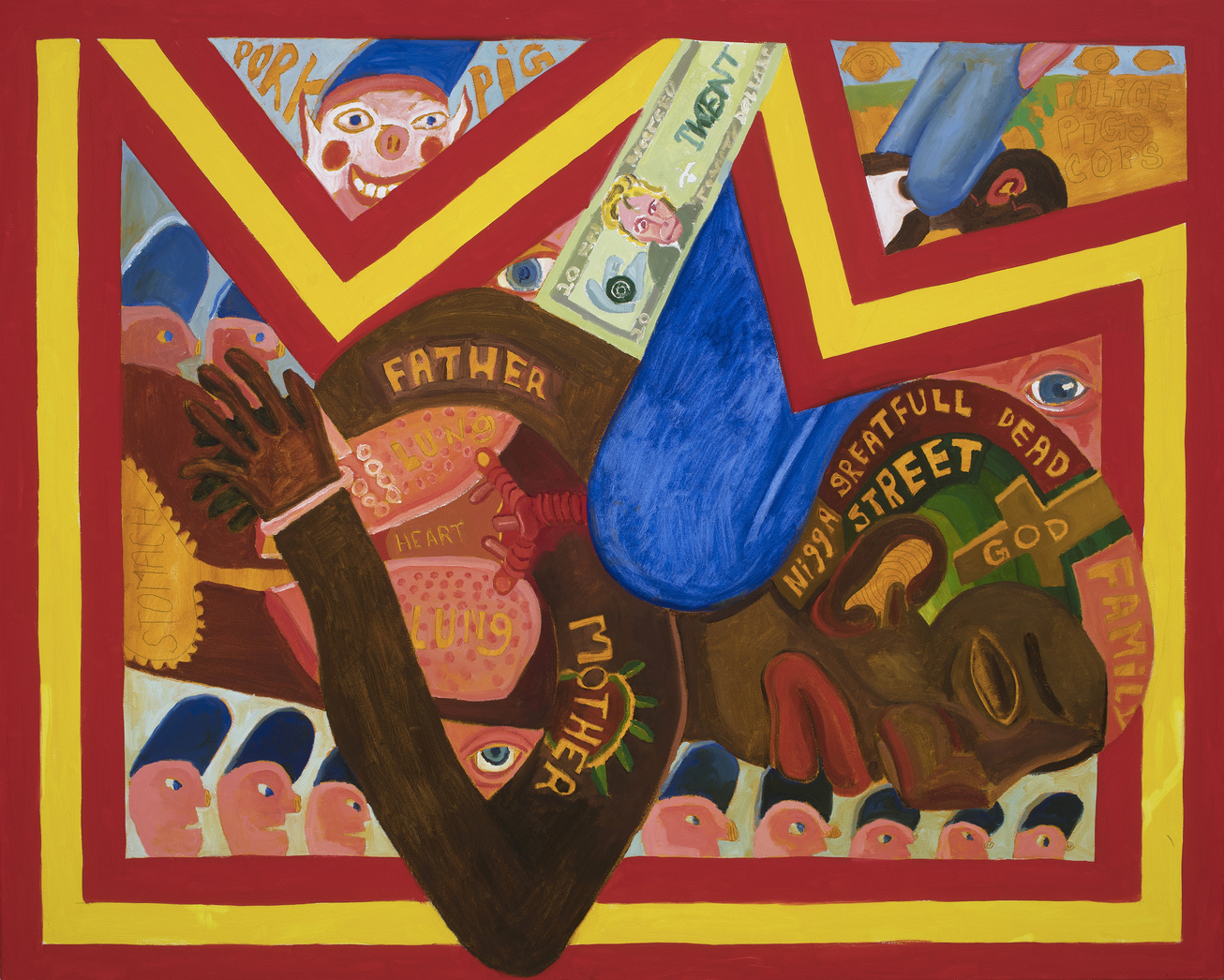This abstract modern art painting features a poignant depiction of a black figure lying down, face toward the bottom, with internal organs such as the heart and lungs visibly detailed. Over the figure's head, various words are written: "Nigga," "beautiful dead," "street," "God," and "family," each in different vivid colors. The arms are marked with the words "mother" and "father." Surrounding the figure, the background bursts with bold red and yellow zigzag patterns.

In the upper left corner of the painting, a crudely drawn pink pig with red cheeks and a blue hat, resembling a clown, is labeled "pork pig." Nearby, an eyeball floats ominously. In contrast, the upper right corner features a disturbing image of a pair of legs kneeling on the shoulders of the black figure, echoing themes of oppression and violence.

Towards the bottom of the piece, a row of pale, pinkish cartoon faces with tall blue hats or hair and mean expressions add to the chaotic atmosphere. Additionally, scattered throughout, there are floating images of a $20 bill, reinforcing themes of materialism and value. A red and yellow border encapsulates the entire artwork, amplifying its intense and provocative nature.